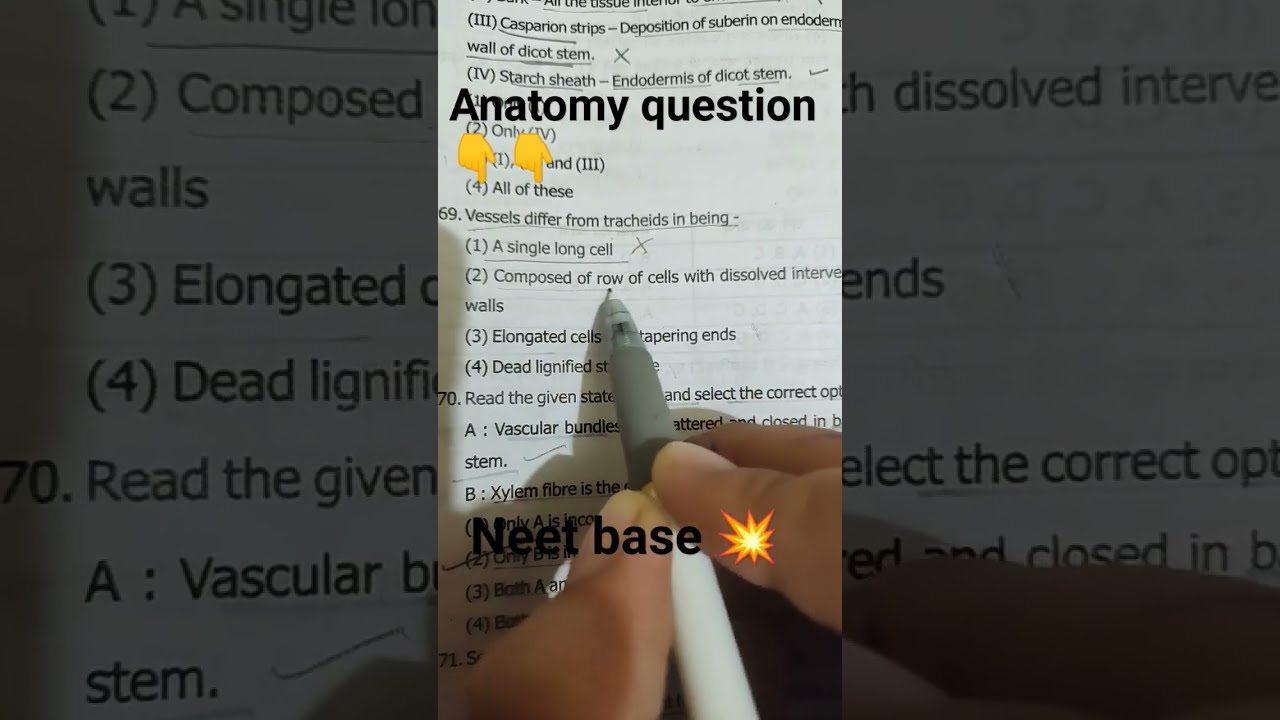The image depicts a page from an anatomy textbook, featuring a complex anatomy question prominently displayed in the center. At the top center of the page, the title "Anatomy Question" is marked in bold, black letters, accented by two yellow emoji hands pointing downward. Below the title is the term "NEET Base" in black text, highlighted by a yellow sunburst emoji. The left and right thirds of the page fade into a dark gray shade, hinting at the text on subsequent pages beneath.

The central portion of the page is lighter, drawing attention to a close-up view of the content. A hand, likely belonging to a student or instructor, holds a pen directed at a specific sentence on the page. This sentence, part of a number-labeled list, includes technical terms like "rows of cells with dissolved walls." Other scientific terms scattered across the page include "Dicot System," "Starch Sheath," "tracheids," "elongated cells," and "vascular bundles."

The detailed image implies an academic setting, possibly someone examining or answering the question, with the intricate anatomical terms underscoring the specialized nature of the content.